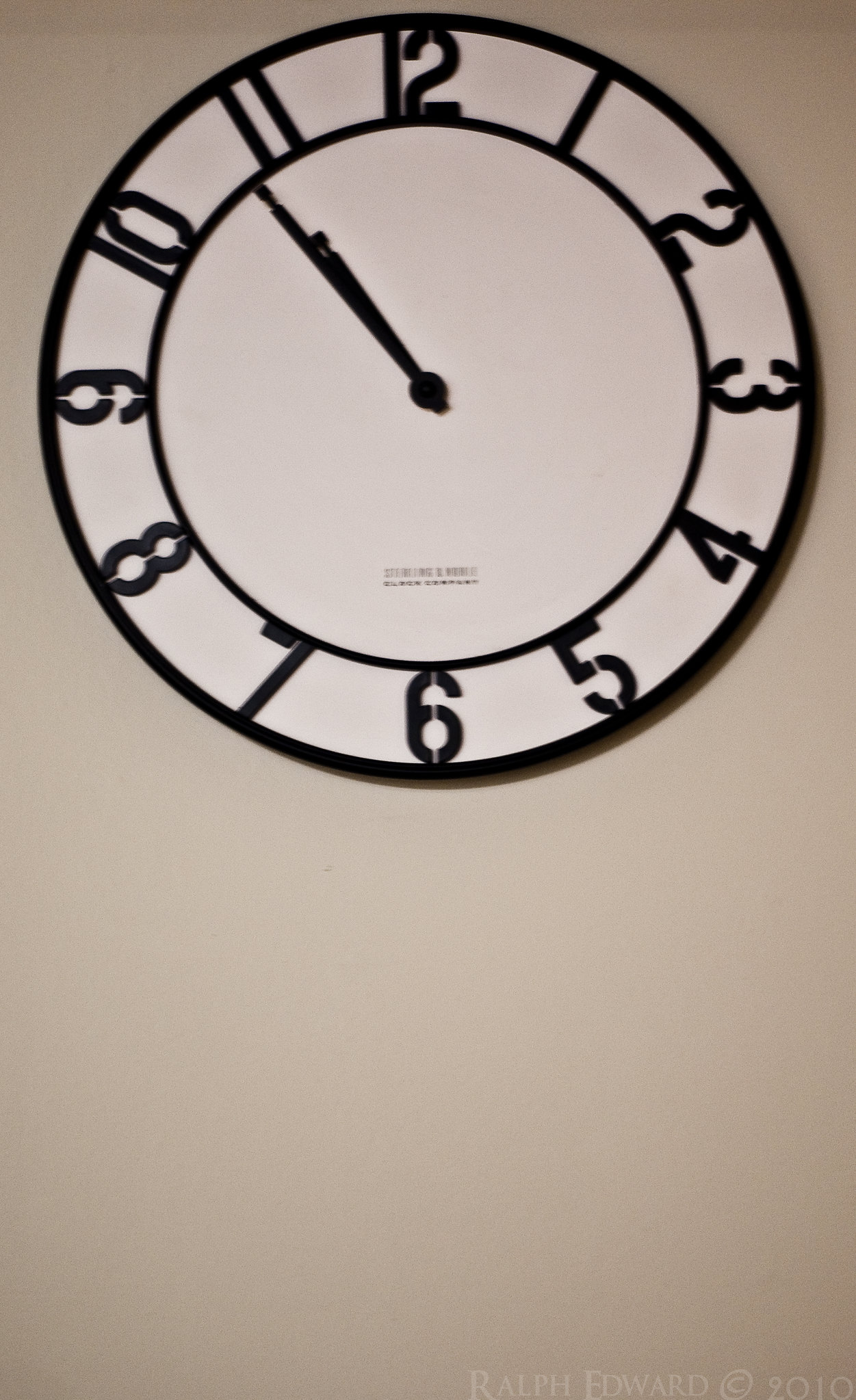The image features a circular, minimalist wall clock set against a light tan wall. The clock, positioned in the top third of the photograph, contrasts sharply with the plain wall that occupies the lower portion of the image. Designed with a modern aesthetic, the clock has a sleek black outer edge and clear, traditional numbering from 1 to 12. The black hands of the clock are positioned to display the time as 10:54. Just above the 6 o'clock marker, the inner face of the clock bears some lettering, likely indicating the manufacturer's name. The overall composition of the image highlights the clock's understated elegance and the simplicity of its surroundings.